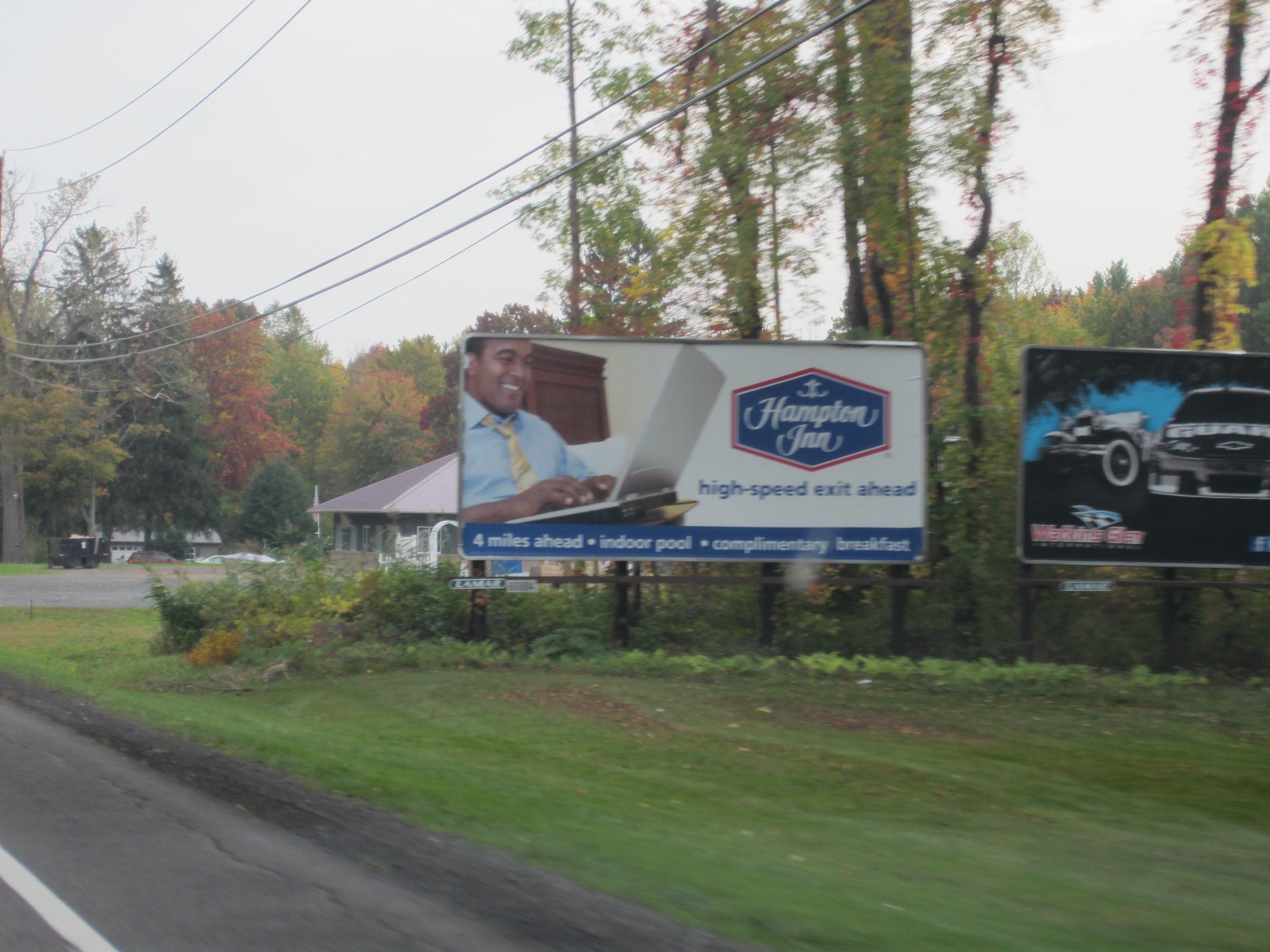Two billboards are prominently displayed along a roadside. The first billboard advertises Hampton Inn, featuring a man in a blue collared shirt and yellow tie using a laptop. The text promotes amenities such as a high-speed exit four miles ahead, an indoor pool, and a complimentary breakfast. The second billboard displays an image of a truck. Below the billboards, a street runs parallel to a grassy area bordered by trees and various plants. In the vicinity, there are two houses visible, one closer to the foreground and the other slightly further back. Additionally, two recycling bins are positioned near the street. The trees in the scene have lush green leaves, with one tree showcasing vibrant red leaves, adding a touch of autumnal color to the landscape.